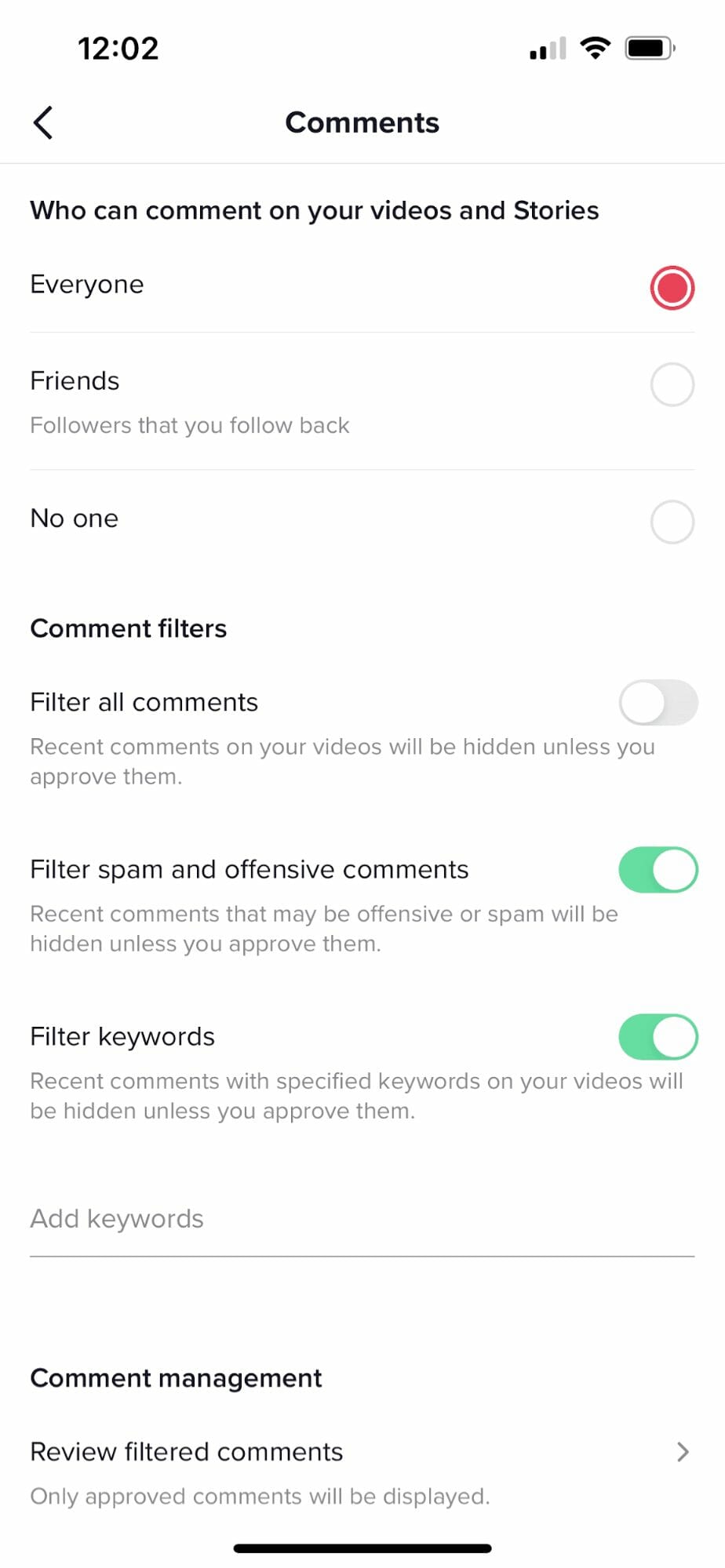The image is a screenshot of a settings pop-up from an application. At the top, it features the title "Commons" prominently. In the upper left-hand corner, the current time is displayed as 12:02. In the upper right-hand corner, several icons are visible: a Wi-Fi indicator showing 2 out of 4 bars, confirming the device is connected to the internet with a Wi-Fi symbol next to it, and a nearly full battery icon indicating the battery is almost at 100% charge.

The main section of the pop-up is titled "Commons" in bold and centered text. Below this title, there are options related to comment permissions on videos and stories. The options are listed as:
1. "Everyone" - This option, highlighted in red, is currently selected as the default.
2. "Friends" - This indicates followers that the user follows back but is not selected.
3. "No One" - This is also not selected.

The next section in the pop-up is labeled "Comment Filters," which includes three toggle sliders for managing comments:
1. "Filter All Comments" - This slider is present but not highlighted.
2. "Filter Spam and Offensive Comments" - This slider is selected, indicating it's active.
3. "Filter Keywords" - This slider is also selected, showing it's in use.

Overall, the settings allow for customization of who can comment and apply various filters to control the content of the comments.